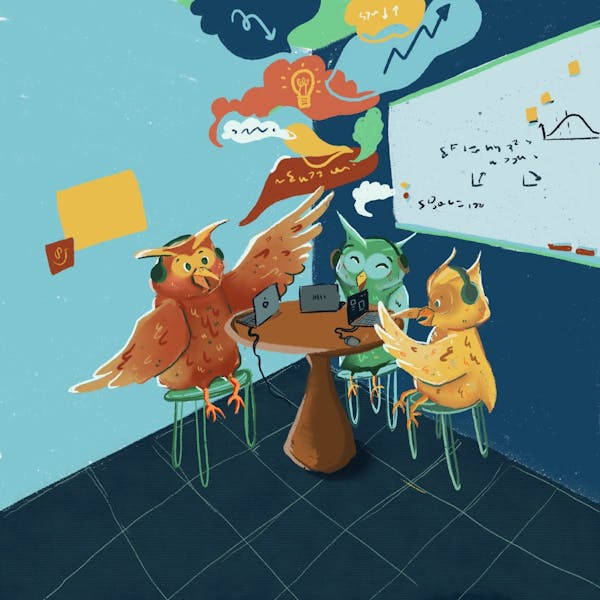This lively illustration depicts three cartoon owls engaged in a brainstorming session at a round, brown table, each equipped with a laptop and headphones. The scene is set in an environment filled with vibrant colors, predominantly featuring shades of blue on the walls and floor tiles. The owls, each uniquely colored in brown, green, and yellow, are seated on green chairs, immersed in their collaborative effort. Behind them, a whiteboard covered with mathematical formulas hints at a scientific or academic endeavor. Surrounding the whiteboard are colorful speech bubbles and arrows in blue, red, and brown, emphasizing the dynamic exchange of ideas. The owl on the left appears particularly animated, with a flurry of speech bubbles suggesting he's leading the discussion, while the others are smiling and contributing enthusiastically. The overall composition captures a harmonious blend of warm and cool tones, projecting an atmosphere of energetic teamwork and intellectual discourse.